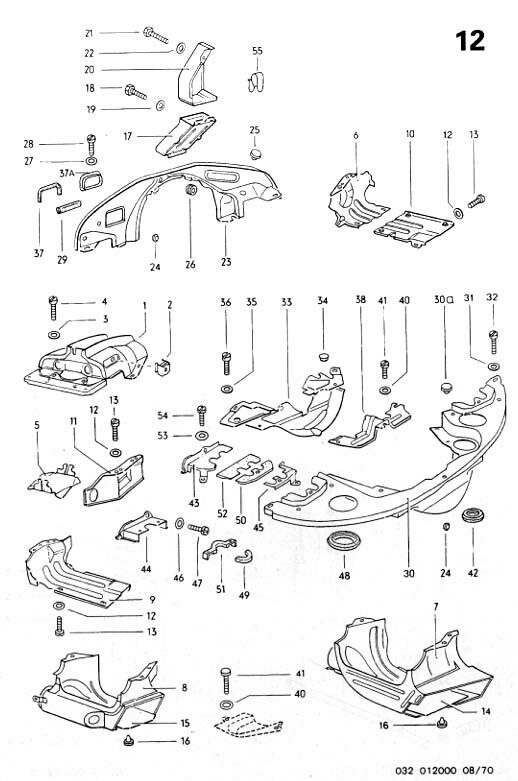The image is a detailed black and white illustration, likely a page from a manual, showing over 50 different mechanical parts, including screws, rivets, washers, and various metal components. Each part is meticulously numbered, resembling the style of assembly instructions, without any names, just numbers. The illustration is marked as page number 12 at the top, indicating its sequence in the manual. Additional specific numbers, "032 012000 08/70," are present in the lower right corner, possibly referencing a catalog or parts number. The layout is designed to guide the assembly or reassembly of what appears to be a car part, potentially a bumper, with lines connecting numbers to each corresponding component.